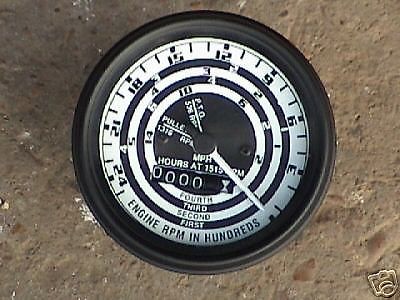This image depicts a detailed close-up of a black thermostat gauge. The central focus of the photograph is the dial that features measurements labeled "Engine A/M" in increments of hundreds. Surrounding the central portion of the dial are several concentric rings. The outermost ring is black, followed by a more prominently extruded black ring. Inside this, there is a white ring that is segmented with numerical markings at intervals ranging from 6, 9, 12, 15, 18, 21, and 24, accompanied by tick marks corresponding to these numbers, likely indicating pressure measurements.

Within this calibrated white ring, there is another black ring that contains additional white marks, albeit indistinguishable in the image. Further inwards, another white ring is present, encircled by another black ring immediately surrounding the central display area.

At the very center is a black circular section, featuring a white, clock-like gauge needle. This needle is connected to a black nozzle-like structure. The entire device rests upon a textured ground, which appears rough and is not fully discernible in detail.